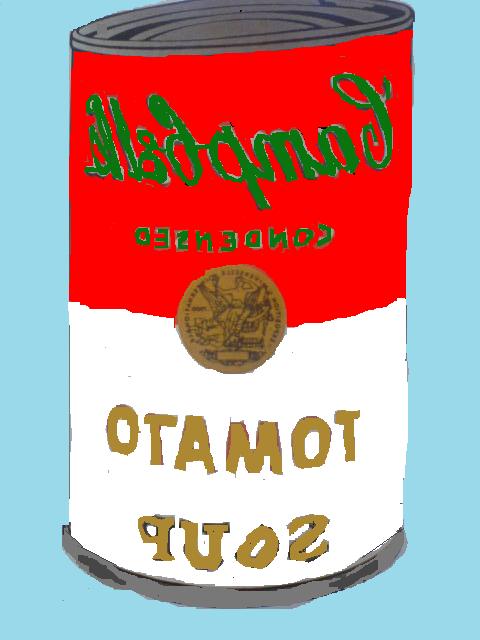This vibrant image showcases a can of Campbell's Condensed Tomato Soup with a striking and unconventional twist. The label, typically familiar to many, is rendered in a distinct pop art style with a rich blue background. The top half of the label features the iconic Campbell's branding in a deep red, while the bottom half is in a clean white. Intriguingly, the text "Campbell's Condensed Tomato Soup" is displayed in a shimmering gold or bronze hue, but it is all written backwards, adding a surreal, reflective quality to the artwork. This imaginative piece appears to be an homage to renowned American pop artist Andy Warhol, known for his famous Campbell's Soup Can series, but with an innovative and playful reinterpretation.